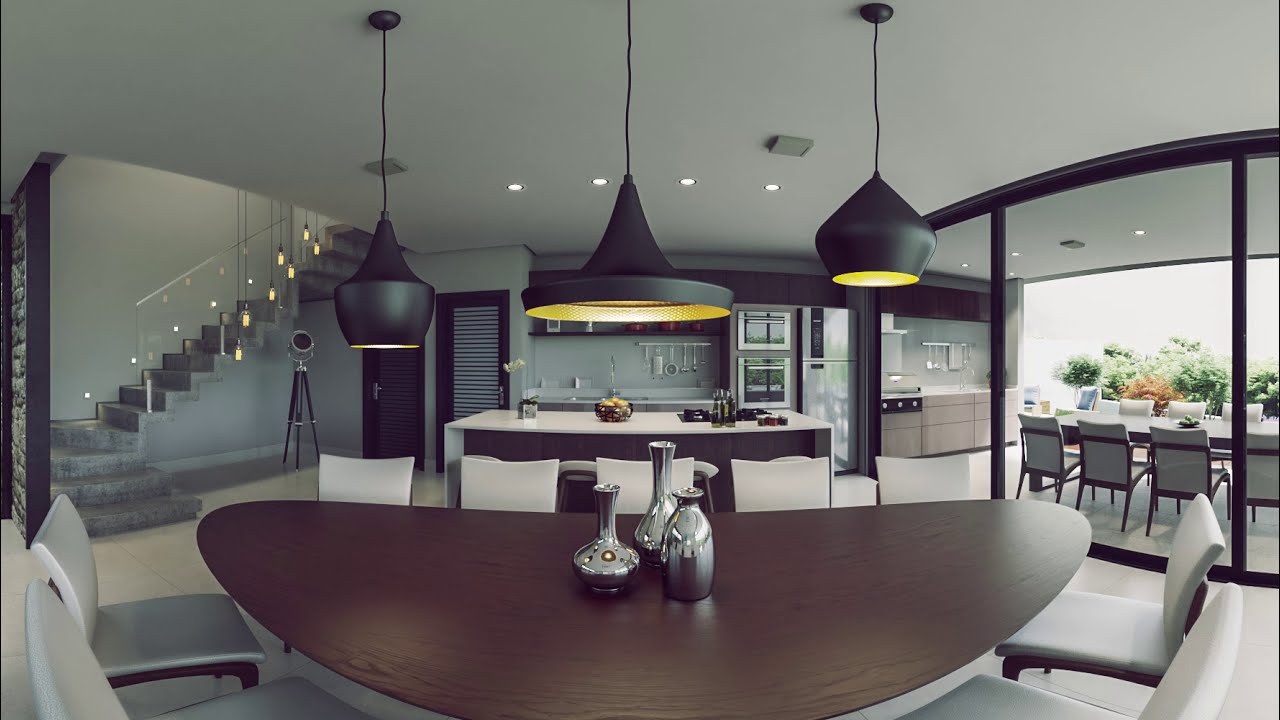The image depicts a beautifully designed, modern kitchen and dining area, possibly a computer-generated rendering. In the foreground, there is a circular dining table with a dark brown top, surrounded by nine white chairs with straight angles, white cushions, and backs. The table centerpiece features three silver vases of various shapes and styles. 

Behind the dining table is a kitchen island equipped with a sink and adorned with a fruit basket and other miscellaneous items. On the adjacent wall, there's a rack holding various kitchen tools, including a strainer, cleaver, and meat tenderizer. Above the island, three black pendant lamps with yellow lighting hang from the ceiling, arranged with two in a teardrop shape and the center one resembling a witch's hat.

To the left of the island, there is a staircase with a gray base and a white glass railing leading to an upper level. To the right, the kitchen opens into a spacious and well-lit seating area with large windows. The windows reveal either an additional seating area or a reflection from within, featuring chairs of the same style as those around the dining table. The area includes a countertop with various bowls and jars and continues towards a space that appears to be a covered patio, also furnished with white chairs and a table. The kitchen ceiling is white, complemented by recessed white lights, enhancing the bright and airy atmosphere.